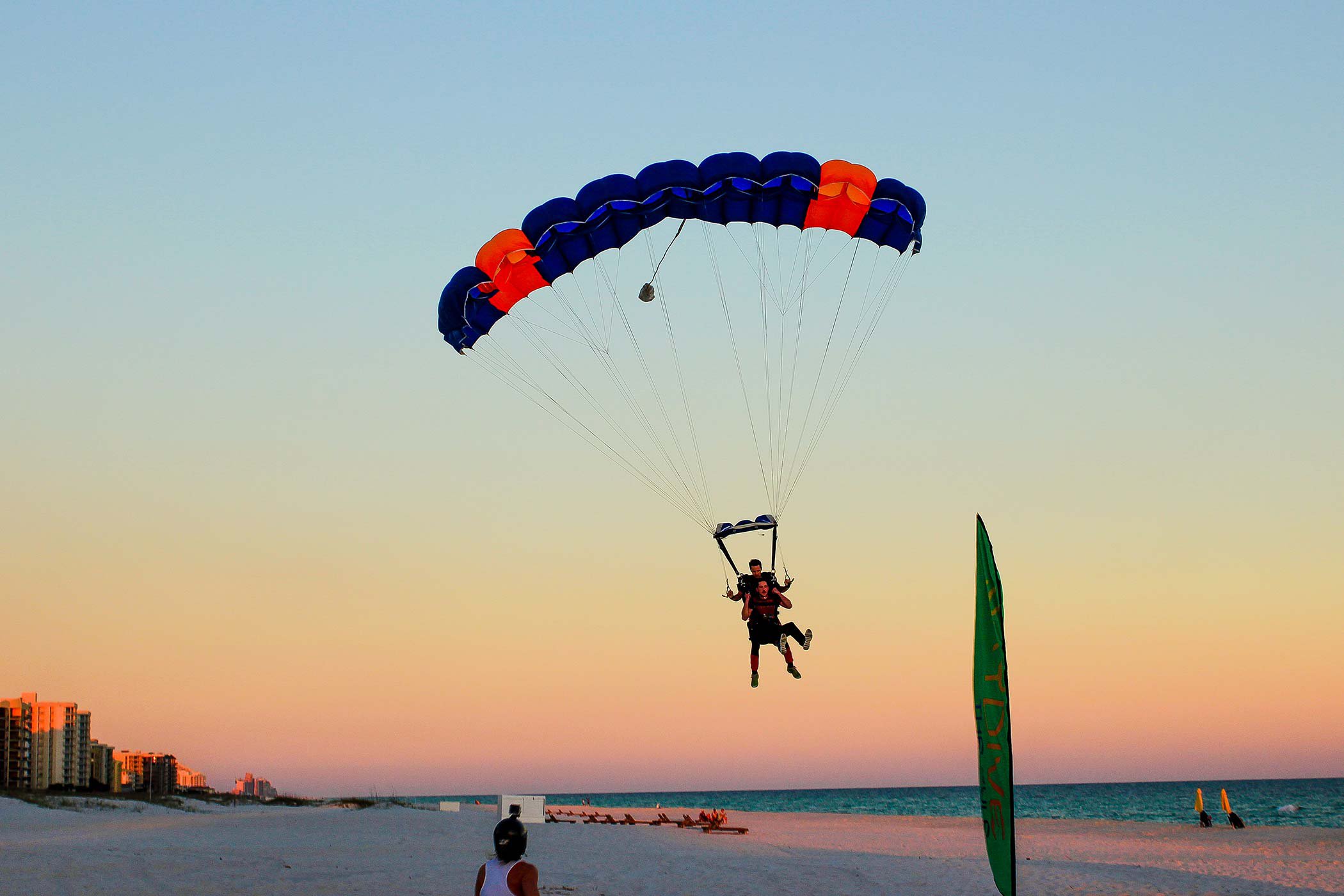This photograph captures the final moments of a tandem hang gliding episode at dusk on a sprawling, sandy beach possibly located in Florida or South America. Dominating the upper part of the image is a striking sky, tinged with hues of pink and blue as the sun sets. Below, the vast beach stretches far, dotted with footmarks and a variety of lounge chairs scattered around. To the left, the horizon features tall buildings, reminiscent of apartment complexes and hotels, while to the right, the serene expanse of the ocean meets the sky.

In the foreground, two individuals are about to touch down, suspended just a few feet above the sand under a blue and orange parachute. The rear person, presumably the pilot, grips the control handles, guiding their descent. Nearby, a surfboard juts out vertically from the sand, and another person stands on the beach, looking up at the gliders. The overall ambience of the photograph conveys a tranquil yet slightly desolate coastal scene, with just a few beachgoers scattered around and the day transitioning into night.